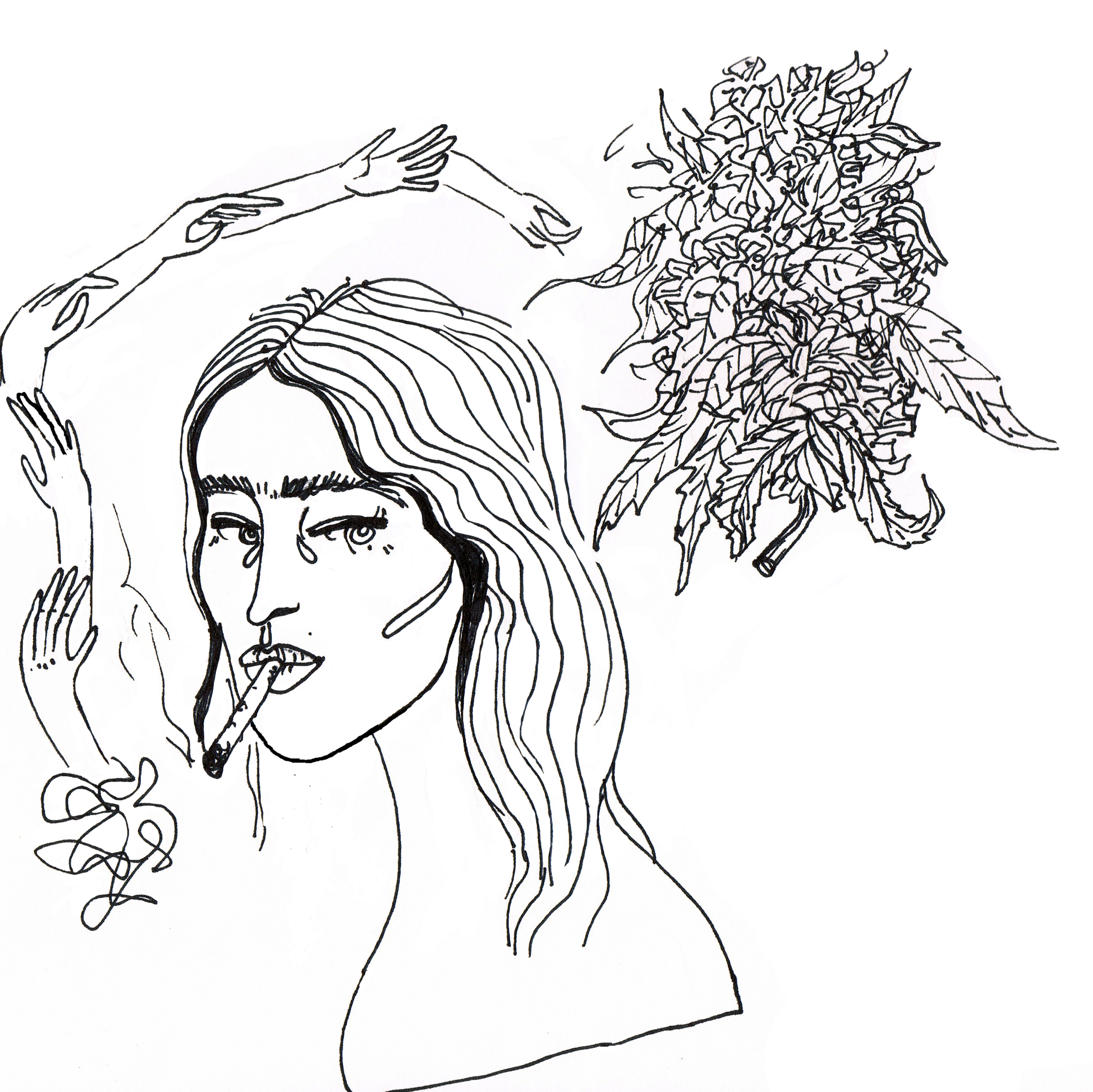The image is an abstract pink sketch primarily done in black ink, capturing the portrait of a young woman from the shoulders up. She has shoulder-length, slightly wavy hair parted in the middle, thick eyebrows, and fairly big lips. Her makeup is dark, and she looks like she has tears forming in the corners of her eyes. A hand-rolled cigarette or joint dangles from her closed lips, with smoke swirling away from it.

The background features a dense cluster of long, random leaves on the upper right side, suggesting cannabis leaves. In front of the woman, there are six disembodied hands, illustrated from the wrists upwards, curving over her head from her chin to the back of her head, intertwined with the smoke emanating from her mouth. The intricate combination of these elements creates a layered, mysterious, and surreal composition.